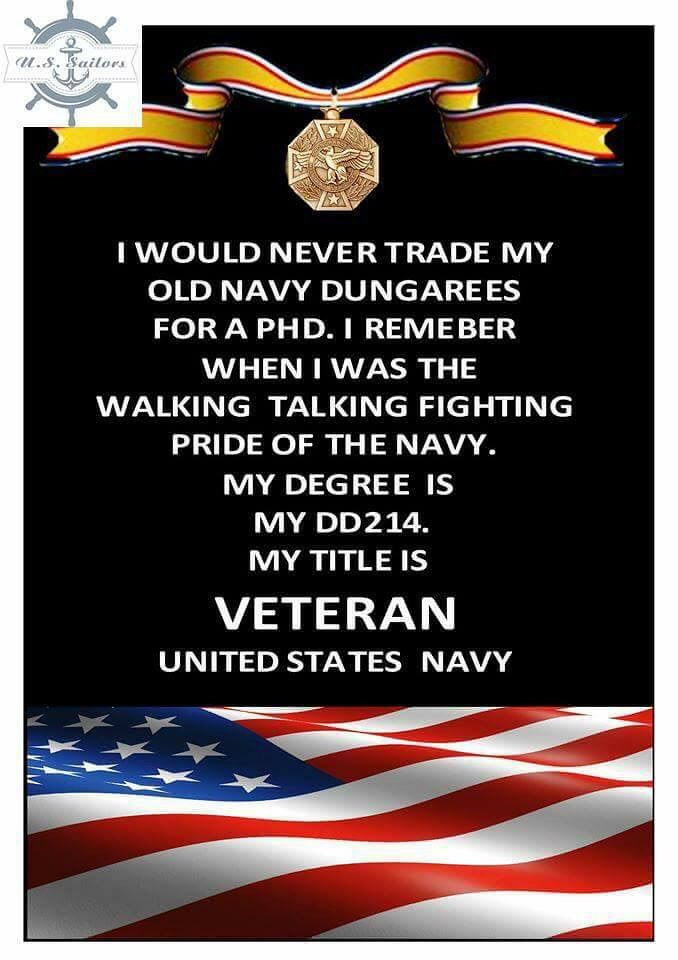The image features a black background with an intricate yellow ribbon at the top, holding a gold medal adorned with an eagle. The medal displays cardinal stars and a diamond design with a green ribbon attached above. In the upper left corner, the text "U.S. Sailors" appears alongside a ship's wheel logo. Central to the image is the prominent text: "I would never trade my old Navy dungarees for a PhD. I remember when I was the walking, talking, fighting pride of the Navy. My degree is my DD214. My title is veteran, United States Navy." Below this text, a graphic illustration of an American flag appears, depicted at an angle.